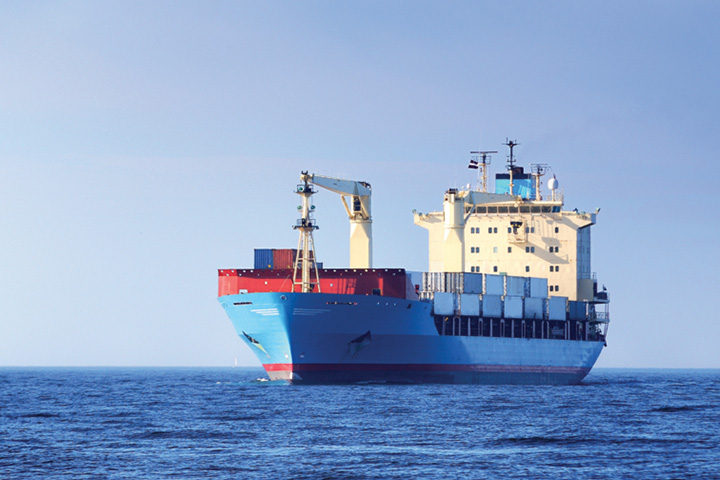The photo captures a large cargo ship gliding across a calm, dark sea under a clear, light blue sky. The ship is predominantly painted blue with a red line along its hull, and is loaded with red shipping containers. Prominent on the vessel is a white crane and a white superstructure towards the stern, which likely serves as an operations area and living quarters for the crew. The bright, sunny day enhances the vibrant colors of the scene, making it a striking image of maritime transportation. Details like the black antenna on the superstructure add to the intricacy of the ship's design. The vessel appears to be a substantial freighter, emphasizing its role in transporting cargo across the ocean.